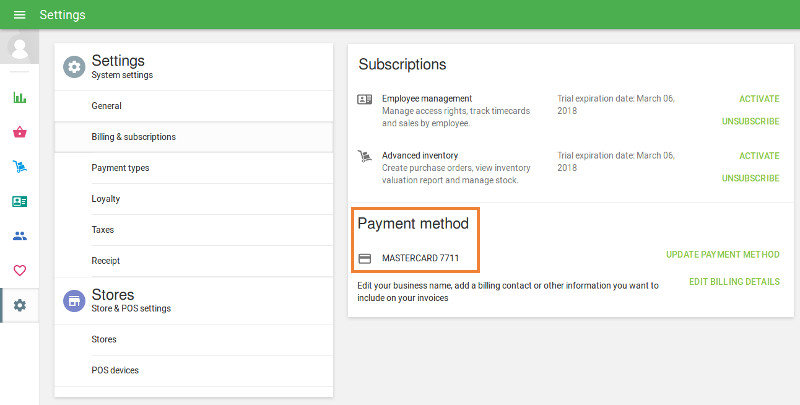The image showcases a computer settings menu with a green bar across the top. On the left side of the bar, there are three white horizontal lines stacked vertically, followed by the word 'Settings' in white. Down the left side of the screen is a vertical task bar. At the top of the task bar is a square space meant for a profile picture, currently empty. Below this are icons representing a graph, a shopping basket, and two other items that are not clearly identifiable. Further down are icons for two people, a heart, and a settings icon, with the settings currently selected.

The main settings column to the right of the task bar displays several categories: 
- System Settings
    - General
    - Billing and Subscription
    - Payment Types
    - Loyalty
    - Taxes
    - Receipts

- Stores
    - Store and PO Settings
    - Stores and PDS Devices

Next to this column is a large rectangle labeled 'Your Subscriptions,' and beneath it, highlighted by an orange square, is the ‘Your Payment Method’ section. This area contains details about subscriptions, employee management, and advanced inventory. Additionally, there are options to edit the business name and add a billing contact.